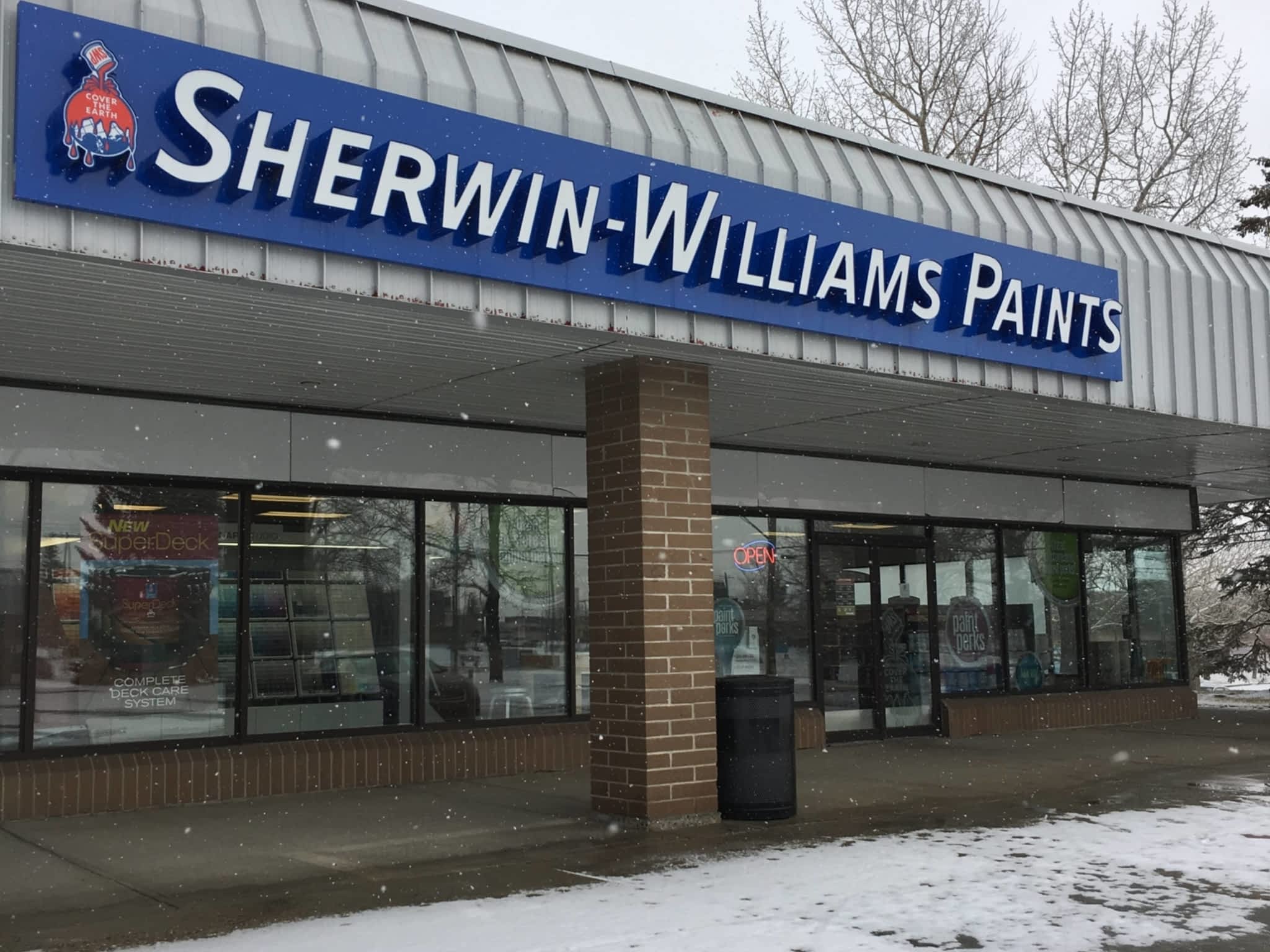This photograph captures the exterior of a Sherwin-Williams paint store during the winter season. The storefront is adorned with the "Sherwin-Williams Paints" name in bold white font set against a rich blue background. To the left of the store's name is the company's iconic logo – a globe enveloped by red paint. This prominent sign is situated above the entrance.

The building's facade is gray and features vertical lines, complemented by a matching gray awning. In the center of the structure, a striking red brick column adds a contrasting element to the design. The windows of the store reflect the parking lot in front, revealing clear images of parked cars, snow-covered ground, and bare winter trees. The reflections are so vivid that the interior of the store remains hidden from view.

On the lower right-hand side of the image, the parking area is dusted with snow, emphasizing the wintry setting. In the upper right-hand corner, the pale blue sky peeks through, dotted with the silhouette of tree branches, some possibly dusted with snow. The overall scene suggests the store could either be a standalone building or part of a strip mall, with ample parking space available for customers.